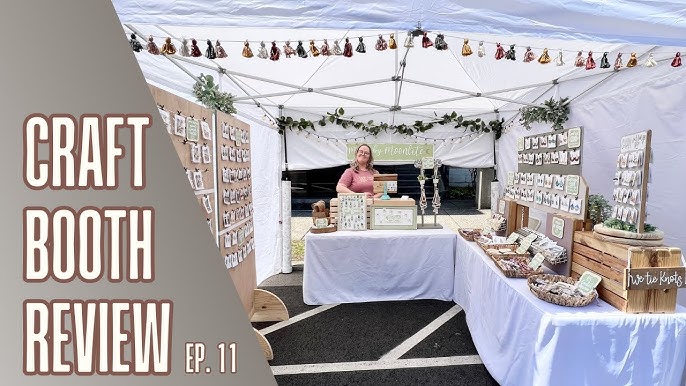A vibrant craft booth is set up under a white exhibit tent in a parking lot, with a black rug and white parking lot lines visible beneath. On the left side of the image, there's a gray triangular area with bold white capital letters outlined in brown that read, "CRAFT BOOTH REVIEW, EPISODE 11." Central to the booth’s setup is a friendly woman wearing a pink shirt and glasses, smiling as she stands at the back. She is behind a table draped in white cloth, forming an L-shape with another longer rectangular table also covered in white drapes to the right, both laden with various craft items and jewelry. The booth is bustling with displays: to the woman's left, a tall wooden board showcases products clipped in rows, and additional pieces hang across the booth on strings and green garlands. Tassels adorn the top of the tent, adding a festive touch. The setup exudes a warm, inviting atmosphere, ready to inform and engage visitors with an array of beautifully crafted items.